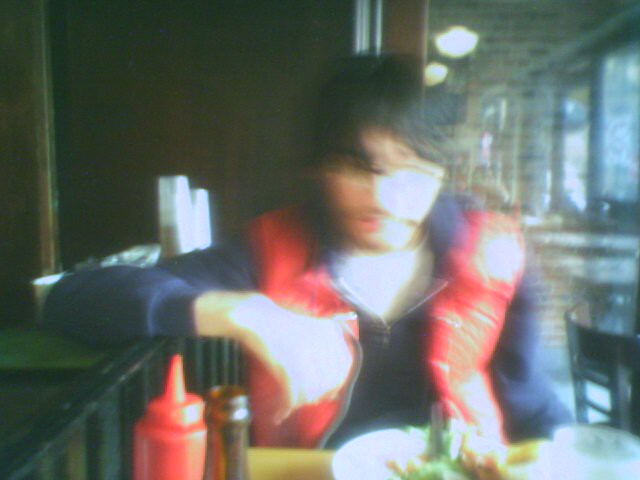This image captures a man seated at a restaurant, though the photograph is extremely blurry. The man appears to be light-skinned and possibly of Asian descent. His black hair is parted to his left side (viewer's right) and falls slightly long. He is dressed in a blue sweater featuring a zipper running from mid-chest to the neckline, topped with a puffy red vest. The man also dons a pair of glasses. In front of him on the table sits a plate of food, though the details of the meal are indiscernible. Additionally, there are two bottles on the table; one is clearly a bottle of ketchup, while the other bottle is unidentifiable due to the image’s blurriness.